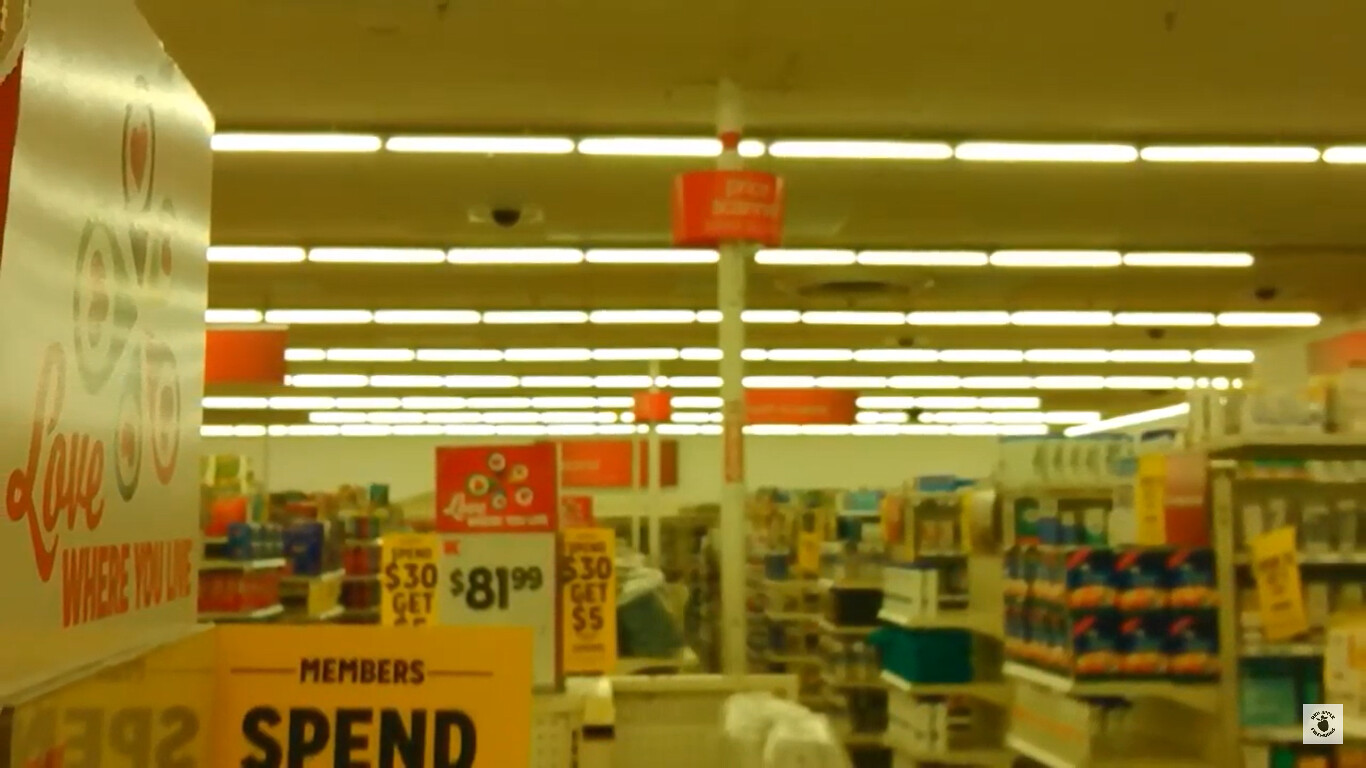The photograph, slightly blurry, captures the lively interior of a grocery store. Dominating the foreground are several signs that draw immediate attention. The most prominent is an orange sign with black text reading "Members Spend." Just behind it, a sign displays a price of $81.99 in black text on a white background, topped by a red sign providing additional details. On the opposite side, you can see two orange signs promoting a deal, "$30 get $5," though the text is partially obscured.

To the far left, there's a white sign angled towards the entrance, reflecting light. It features red cursive text that reads, "Love," with "where you live" written below, offering a charming welcome as customers enter. Despite the multitude of signs, the store appears meticulously organized and the shelves fully stocked, resembling a discount outlet like Big Lots, Kmart, or T.J. Maxx, yet maintaining an inviting and pleasant atmosphere.